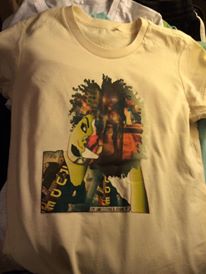In the photograph, we see a stack of t-shirts, with the top one prominently displayed. This top t-shirt is yellow with a crew neck and distinctive design. The design features an ethnic-looking woman with an afro of very curly hair, her head tilted slightly to the side, and she is looking off to the left with her eyes. The image on the t-shirt is vibrant and colorful, with the woman's skin depicted in varying hues of greenish-yellow and lime green. Her lips are dark green, and within her hair, there are striking colors such as orange, green, and purple. The shirt she is wearing in the design has black elements and indecipherable letters. Behind this vibrant yellow t-shirt, there is a white t-shirt visible only through its collar, peeking out from underneath. The fabric of the yellow shirt shows some gentle ripples, adding texture to the photograph.